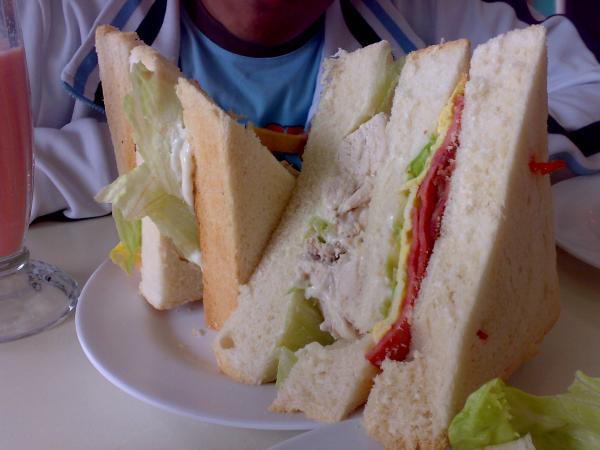This is a highly detailed, close-up photograph of a meticulously presented chicken club sandwich, or perhaps a similar club sandwich, set on a small white plate. The sandwich is cut into two triangle halves, which are standing upright and set opposite each other, forming a striking triangular shape. The sandwich consists of three large slices of white bread, held together by fancy toothpicks, one of which has a red curly tip.

Inside the sandwich, layers of green lettuce, yellow cheese, a slice of red meat, and a light-colored mixture, possibly chicken or tuna salad, are visible. The sandwich appears generously dressed, with mayonnaise visibly spread between the layers. 

The plate is too small for the sandwich, causing the bread on the right side to extend off the plate. To the left of the plate, there is a tall glass containing a pinkish or reddish smoothie-like drink. 

In the background, only the chin and upper chest of a person are visible. They are wearing a blue t-shirt underneath a white track jacket with blue and black stripes on the collar. The person's arms are leaning on the table, adding context to the dining scene. The white countertop further suggests the setting is likely a casual diner.